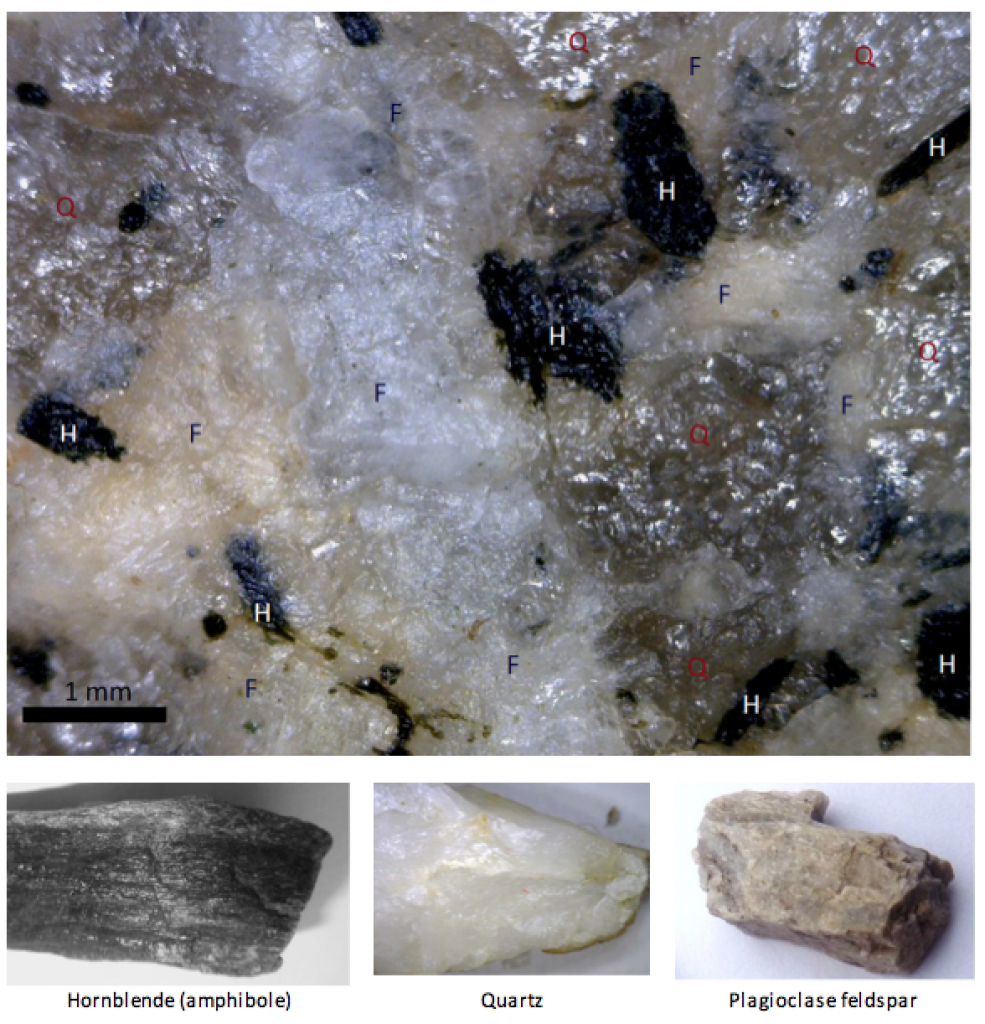This photograph presents a detailed cross-section of a conglomerate rock formation. The top segment of the image depicts this mixed rock with clearly labeled sections, denoted by "H" for hornblende, "Q" for quartz, and "F" for plagioclase feldspar. Hornblende is prominently featured, identifiable by its black, shiny appearance, scattered throughout the image. Quartz, primarily centered, shows as white and glossy, whereas plagioclase feldspar appears as silver-brown, also shiny, located in various areas like the bottom right and top left. The bottom portion of the photograph showcases individual labeled samples of these rocks: on the left is the dark, glossy hornblende, labeled "amphibole"; in the center is the white and shiny quartz; and on the right, the silver-brown feldspar. This detailed imagery and labeling provide a comprehensive visual and educational examination of the rock's composition.